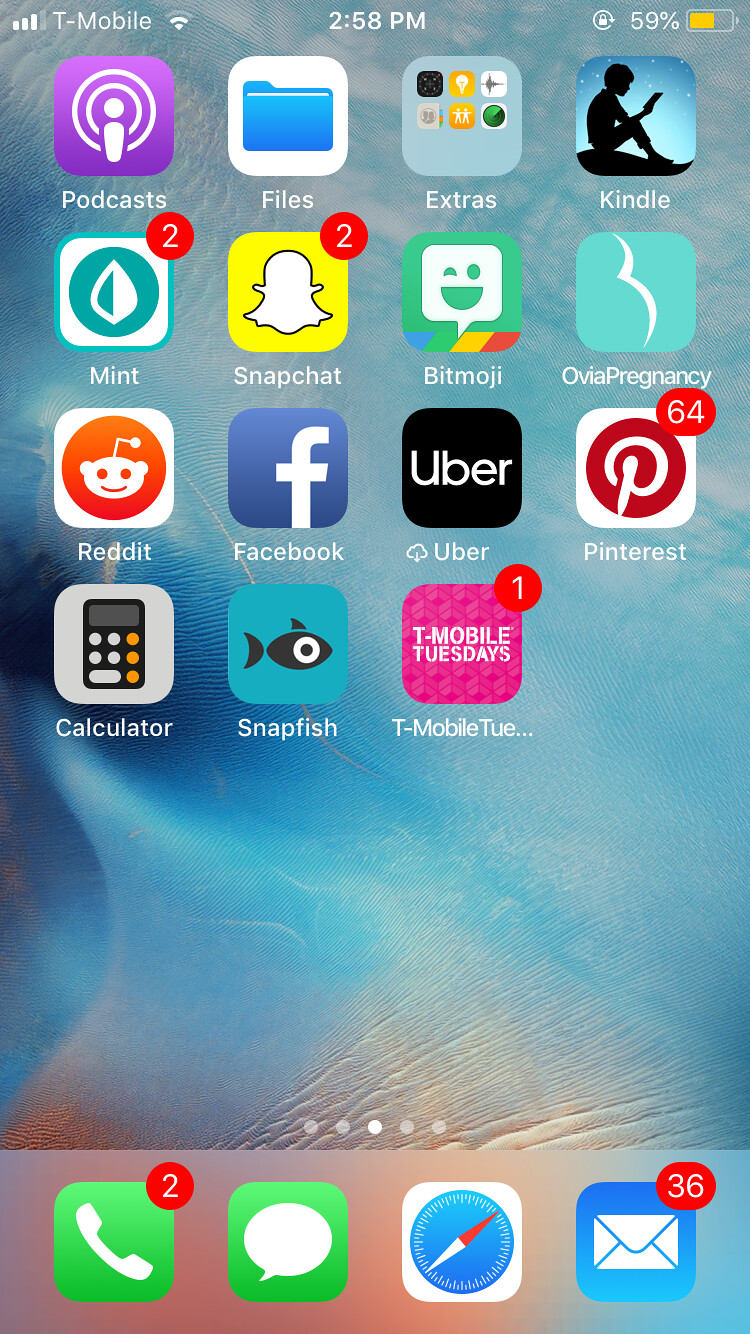This screenshot displays an iPhone's home screen with various details and app notifications. 

**Top Bar Details:**
- **Top Left:** Three signal bars, T-Mobile service provider, three Wi-Fi signal bars.
- **Top Center:** The current time, 2:58 PM.
- **Top Right:** Rotation lock icon, 59% battery life (highlighted in yellow).

**Background:** 
A light blue, abstract ocean-themed image with various hues depending on lighting.

**App Layout:**
- **First Row:**
  - Podcasts
  - Files
  - Extras (folder containing six apps)
  - Kindle

- **Second Row:**
  - Mint (2 notifications)
  - Snapchat (2 notifications)
  - Bitmoji
  - Ovia Pregnancy

- **Third Row:**
  - Reddit
  - Facebook
  - Uber
  - Pinterest (64 notifications)

- **Fourth Row:**
  - Calculator
  - Snapfish
  - T-Mobile Tuesdays (1 notification)

**Dock:**
- Phone (2 notifications)
- Messages
- Safari
- Mail (36 notifications)

This detailed caption provides an exhaustive overview of the iPhone home screen, highlighting the apps, their arrangement, and corresponding notification counts.